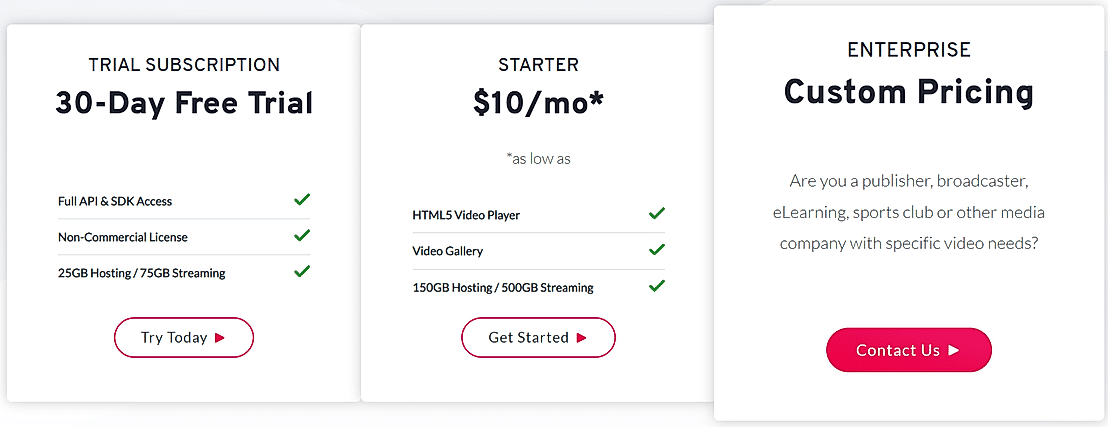**Detailed Caption:**

This image is a detailed screenshot illustrating a tiered pricing structure for a video hosting and streaming service. 

1. **Trial Subscription**:
   - **Duration**: 30-day free trial
   - **Features**: 
      - Full API and SDK access (indicated by green check mark)
      - Non-commercial license (indicated by green check mark)
      - 25 GB of hosting and 75 GB of streaming capacity (indicated by green check mark)
   - **Call to Action**: "You can try it today."

2. **Starter Plan**:
   - **Price**: $10 per month
   - **Features**:
      - HTML5 video player
      - Video gallery
      - 150 GB of hosting
      - 500 GB of streaming

3. **Enterprise Plan**:
   - **Price**: Custom pricing
   - **Target Audience**: Publishers, broadcasters, e-learning institutions, sports clubs, and other media companies with specialized video needs
   - **Call to Action**: "Contact us" highlighted in red text next to a red icon, drawing attention to the need for potential customers to reach out for more information.

The image highlights the salient points of each plan in a clear and organized manner, making it easy for potential customers to compare and choose the option that best fits their needs.